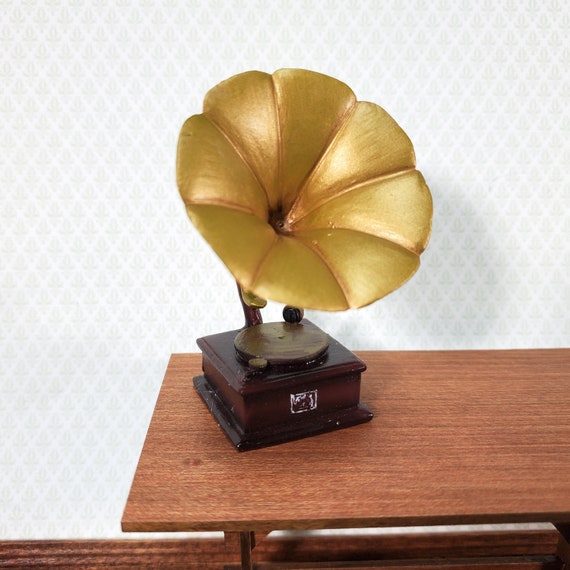This color photograph showcases a miniature, antique-style phonograph, situated atop a wooden table. The background features a white, wallpapered wall with diagonal lines and subtle bluish designs. The phonograph, an unmistakable replica from over a century ago, displays a wooden rectangular base with a markedly shabby appearance, evident from its chipped paint and occasional cobwebs. The base also holds a small circular turntable where a record would traditionally be placed, emphasizing its miniature scale. Dominating the scene is a large, golden, bell-shaped flower speaker, likely metal and gold-plated, designed to mimic the sound projection of a real phonograph. The overall craftsmanship is lackluster, with haphazard and sloppy paintwork contributing to its unattractive aesthetic. A partially obscured metallic square, possibly a logo, adorns the front of the wooden base, adding a touch of historical authenticity to the piece. Despite its detailed components, the phonograph’s unsophisticated finish suggests minimal effort in its creation.